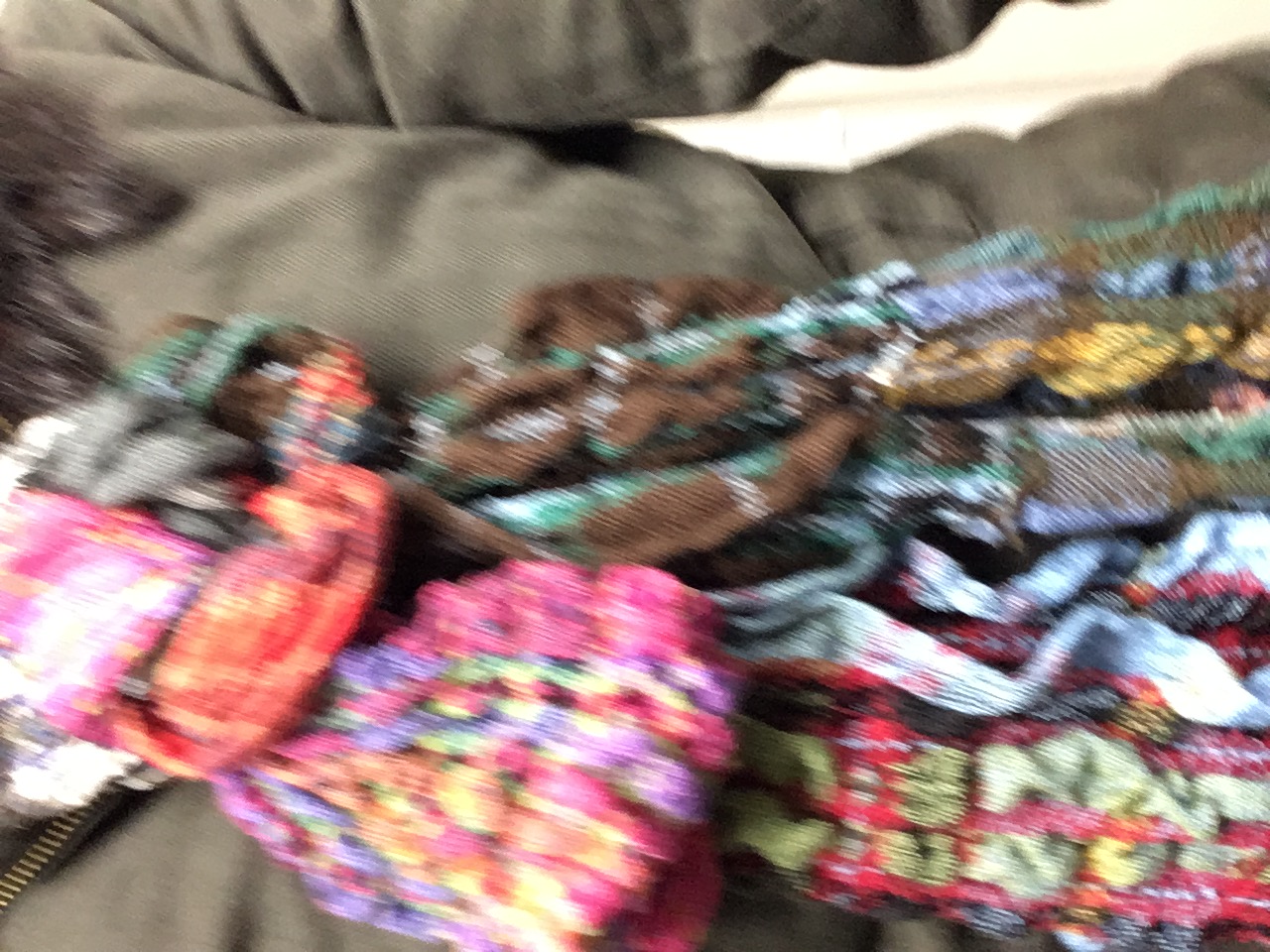The image depicts a blurry photograph of a woman taken from her neck down to her waist, featuring a semi-fitted gray or off-gray jacket that appears to be made of cotton or tweed. She has shoulder-length dark hair cascading down her left side. The most striking detail is her long, multi-colored knitted scarf, which wraps casually and somewhat sloppily around her neck, with colors transitioning from brown, turquoise, and blue on one side to pinks, oranges, purples, greens, and yellows on the other, and finally ending in greens, reds, yellows, and blacks. The overall impression is of a vibrant and textured ensemble captured in motion, though the photograph is extremely blurry and slightly ambiguous in terms of perspective.